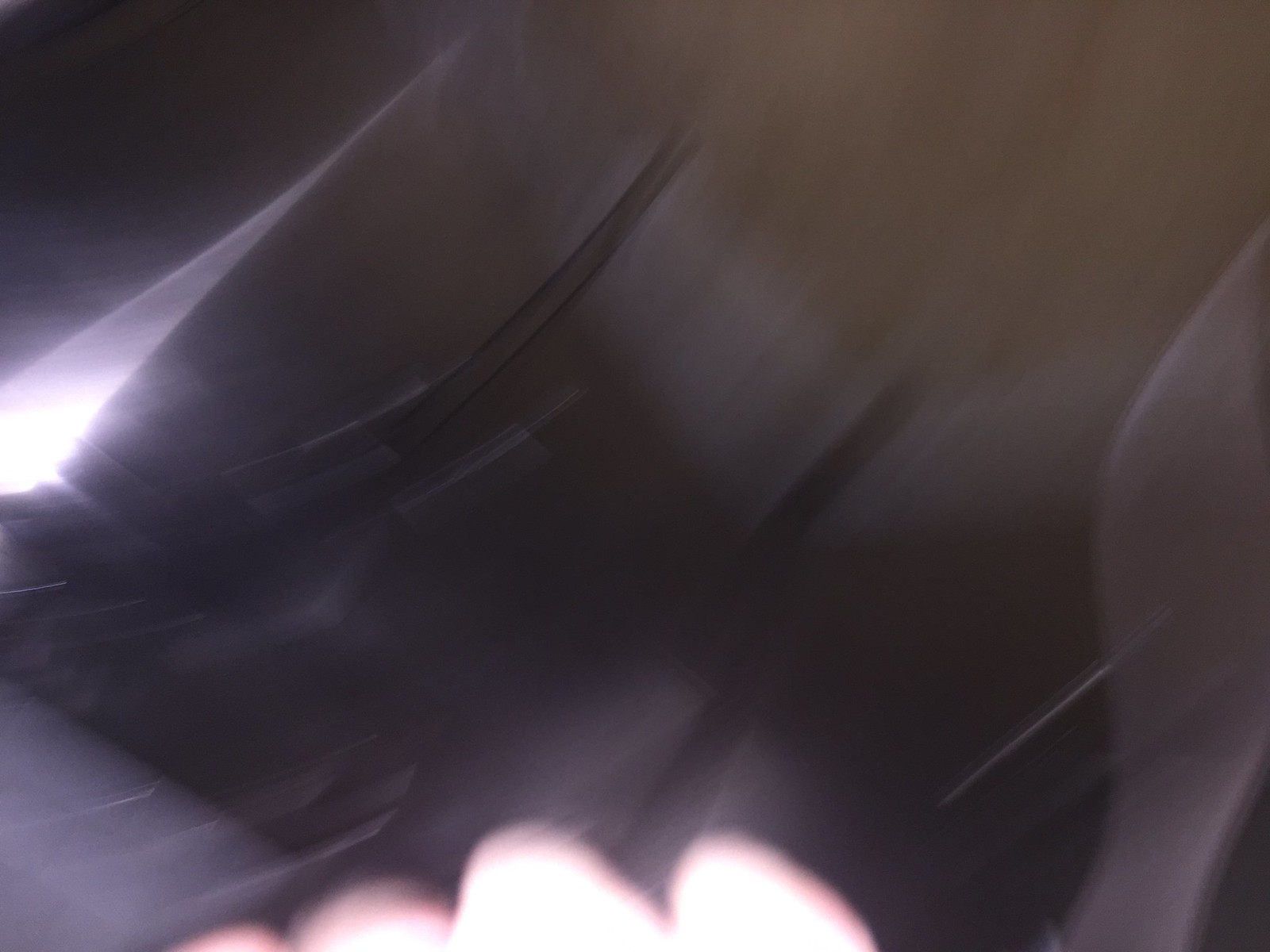The image depicts an abstract scene, dominated by a complete blur that makes specific details indistinguishable. Swirling, curved lines emanate from the left side of the frame, extending upwards but not quite reaching the top. These lines add a sense of fluid motion to the composition. Positioned at the far left center is a bright light or reflection, which arcs diagonally upwards towards the center of the image, creating a focal point. The backdrop transitions from deep black to a brownish-yellow gradient. At the bottom of the image, there are four light-colored, curved semi-circles which could potentially be interpreted as stubby fingers or another undefined object. A lighter strip is visible in the lower right corner, adding a contrasting element to the predominantly dark and abstract background.